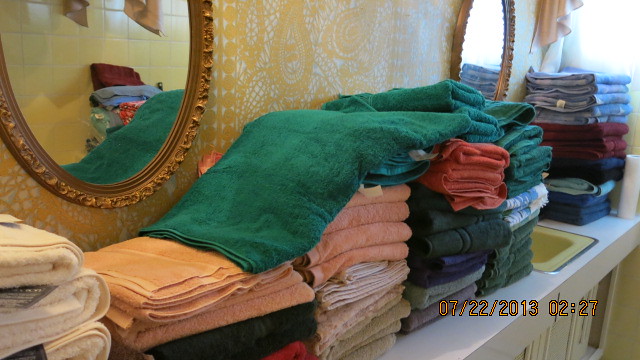The image depicts a long bathroom vanity adorned with an impressive array of towels, meticulously folded and organized by color. The vanity boasts a vast countertop, which though simple in design, serves as the stage for the vibrant display of textiles. Dominating the foreground is a partially unfolded green towel, draping lazily over stacks of orange and tan towels beneath it. To the left, cream-colored towels, still bearing their tags, add a touch of newness to the scene. The towels stretch across the length of the countertop in at least five distinct stacks, each comprising a variety of colors including pink, white, light blue, maroon, and navy blue. In total, the multitude of towels seemingly amounts to about fifty in number. 

Above the countertop, two gold-framed oval mirrors are positioned symmetrically against a backdrop of yellow paisley-patterned wallpaper, reflecting the intricately tiled yellow walls of the bathroom. The vanity features twin gold-trimmed sinks and a small yellow square sink, enhancing the opulent yet serene atmosphere. A towel, possibly hanging in the background, and the meticulous arrangement of folded towels, lend a sense of order and luxury to the bathroom setting.